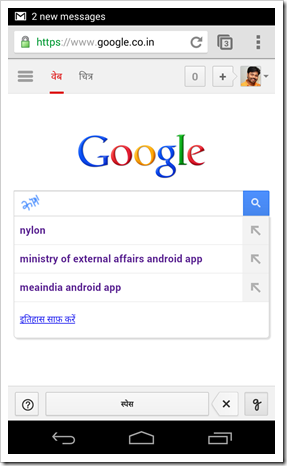This image is a screenshot taken from a mobile device, characterized by its vertical orientation. It features a white border along the top, sides, and bottom, which is just inside of a black frame. On the top left corner, the Google Mail icon is prominently displayed next to the text "2 new messages." 

Below this, the area transitions into a roughly two-inch gray section. At the top of this gray area, a white search bar stretches across approximately two-thirds of the way. It includes a green lock followed by green "HTTPS," then in light gray, several backslashes are present leading to the bold black text "www.theninboldedblack.google.co.in." Near the search bar's end, there is a refresh icon. Outside the search bar, a darker gray border encases a square with a dark gray number "3" in it, followed by three vertical dots.

To the left, there are three horizontal black lines about a quarter of an inch long, followed by red and black Chinese characters. Next to the text, a profile picture of a man in a dark orange shirt is visible on the right side. The area from this section down to the lower two inches of the image features a white background centered around the classic Google logo in its iconic colors. Below the Google logo, a blue search icon is accompanied by text in Chinese scripts. 

To the right, a blue square containing a white search icon is highlighted. Under this section, four clickable drop-down suggestions appear. The top three are in purple text, reading "Nylon," followed by "Ministry of External Affairs," and "Android app." The last suggestion, "me, A-India," is also an Android app, listed in blue Chinese characters. 

The bottom of the image features a gray border containing several symbols: a square with a question mark, a space bar, a square with an "X," and a square with a "G." Finally, the bottom-most part of the screen is black, featuring navigation icons: an arrow for "back" on the left, a home icon in the center, and a white square rectangle on the right.